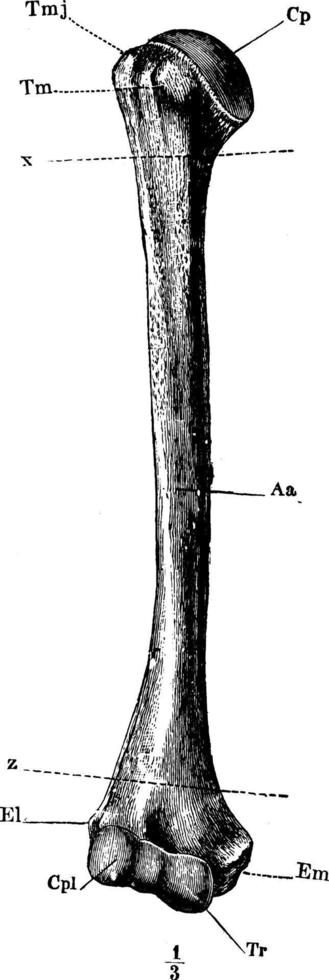This detailed black-and-white drawing depicts a bone, possibly a femur or humerus, though it might belong to either a human or an animal. The bone is oriented vertically with a slight curve near the bottom, where it also widens and resembles the shape of a foot with indentations that evoke toes. The background is left blank, focusing attention solely on the bone itself.

The labeling on the bone is extensive and diverse. Starting at the top, the labels include CP, TM, and TMJ, with a dashed line annotated as X bisecting the upper part. As you move down the shaft, you encounter the labels CPAAEMTR and a distinct marker at the middle labeled "A." Near the lower section, a label "Z" appears just before another dashed line. Below this, the labels EL, CPL, and TR are positioned near what might be considered toe-like features on the bottom of the bone, with the notation "1/3" directly under the bone. Additionally, the letters EM are also present on one of the lower extensions.

The detailed annotations, combined with the clear yet simple monochromatic illustration, suggest an educational or anatomical purpose, making the distinctions and features of the bone easy to study.